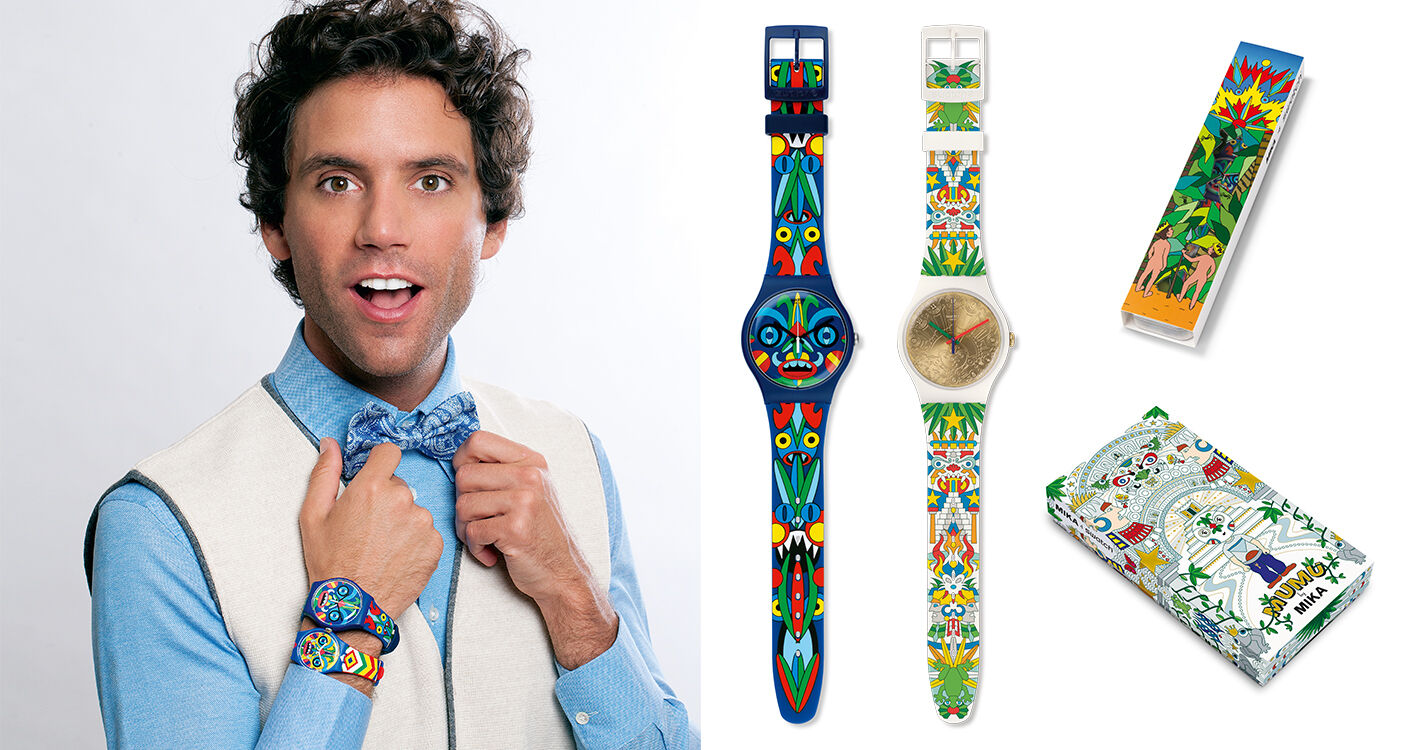This image appears to be a vibrant advertisement for children's watches. It features a rectangular composition with a model on the left side, wearing both watches showcased in the photograph. The model, characterized by brown curly hair, brown skin, and a blue dress shirt paired with a white vest, is striking a confident pose with his mouth slightly open and looking straight at the viewer.

On the right side of the image, two watches are displayed in open, vertical boxes that reveal their full, ornate bands and faces. The first watch has a dark blue backdrop and is adorned with an intricate tribal or indigenous design, featuring stacked tiki-like heads in bright colors such as yellow, red, light blue, and green. The watch face includes a gold hue, depicting one of the tribal faces, and more festive elements like leaves and yellow stars.

The second watch mainly showcases white as its base color, complemented by bold red, green, and blue designs. Its face is golden, adding a touch of elegance, and the band continues the festive tribal theme. Both watches come in multicolored boxes with vibrant tribal patterns, one adorned with an axe and a thick pyramid design, reinforcing the cultural aesthetic.